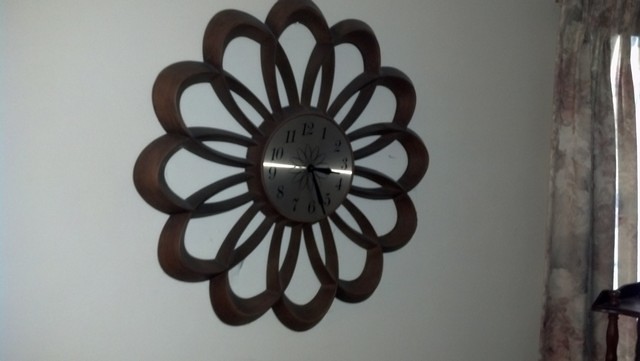In this image, a round wall clock takes center stage with its striking design. The clock face features black hour and minute hands and is adorned with a flower motif that spans the entire face, creating the appearance of a bloomed flower. The numbers 1 through 12 are clearly visible around the clock's circumference. Crafted from dark wood, the clock is mounted on the wall. Adjacent to the clock, floral-patterned curtains frame a window, hinting at a bright and sunny day outside. In front of the curtains, a wooden stand adds to the cozy, homely ambiance of the scene.